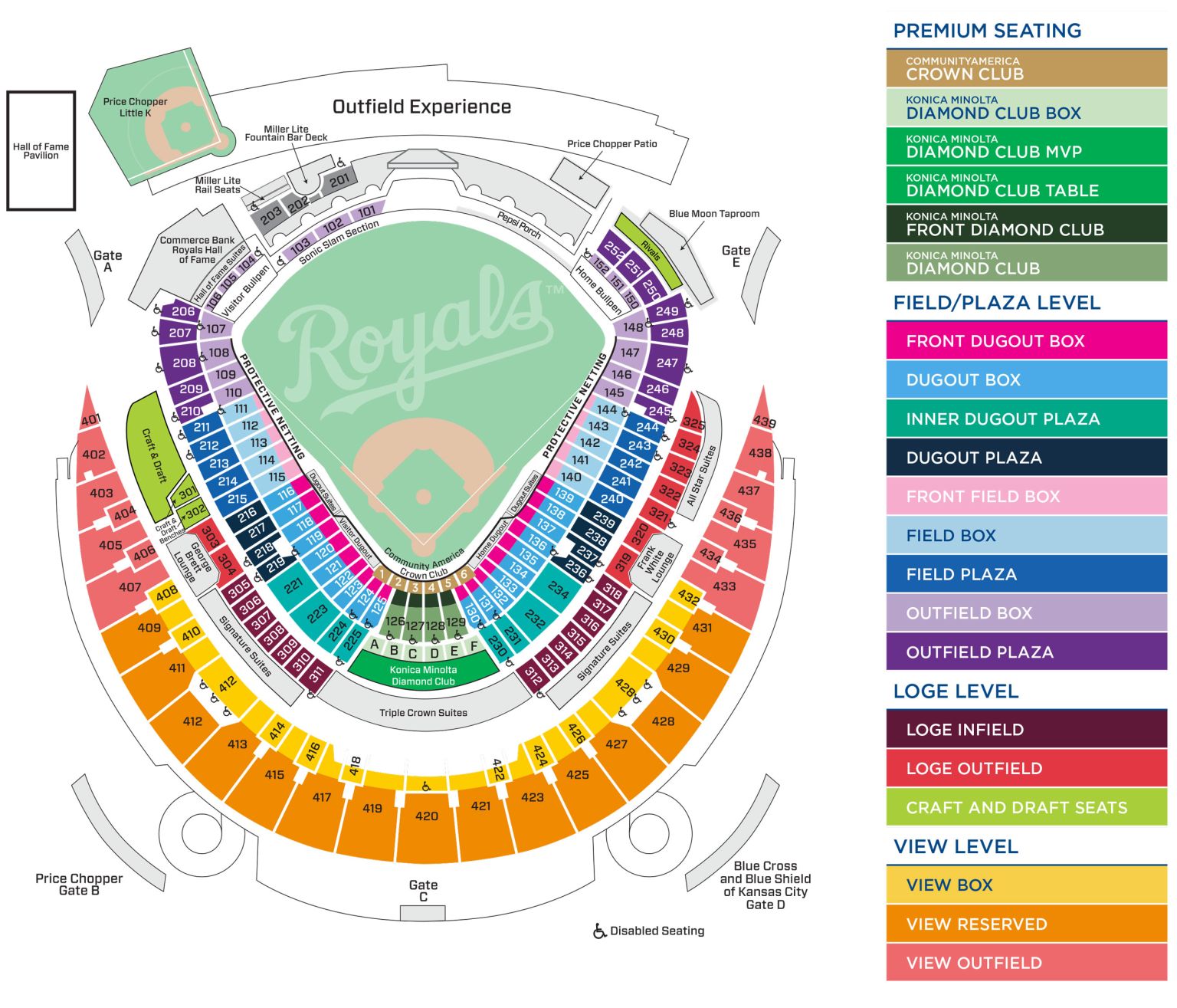Screenshot of Royal Stadium Ticket Map: 

The image displays a comprehensive ticket map for Royal Stadium, divided into two primary sections. On the left, a large white square showcases a detailed map of the stadium, including the ball field prominently labeled "Royals." The seating areas are illustrated in various colors corresponding to their categories.

On the right side of the image, a vertical stack of color-coded rectangles provides a key to the seating areas, each labeled to specify their location within the stadium. At the top portion of the right section, titled "Outfield Experience," the seating categories are listed as follows:

- Premium Seating
- Crown Club
- Diamond Club Box
- Diamond Club MVP
- Diamond Club Table
- Front Diamond Club
- Diamond Club
- Field Plaza Level
- Front Dugout Box
- Dugout Box
- Indoor Dugout Box
- Dugout Plaza
- Front Field Box
- Field Box
- Field Plaza
- Outfield Box
- Outfield Plaza
- Lodge Level
- Lodge Infield
- Outfield
- Craft and Draft Seats
- View Level
- View Box
- View Reserved
- View Outfield

Each category is represented by distinctly colored rectangles, matching the hues used on the stadium map to indicate the respective seating locations. The map provides a complete view of the field and surrounding areas, enabling potential ticket buyers to easily identify and select their preferred seats within Royal Stadium.